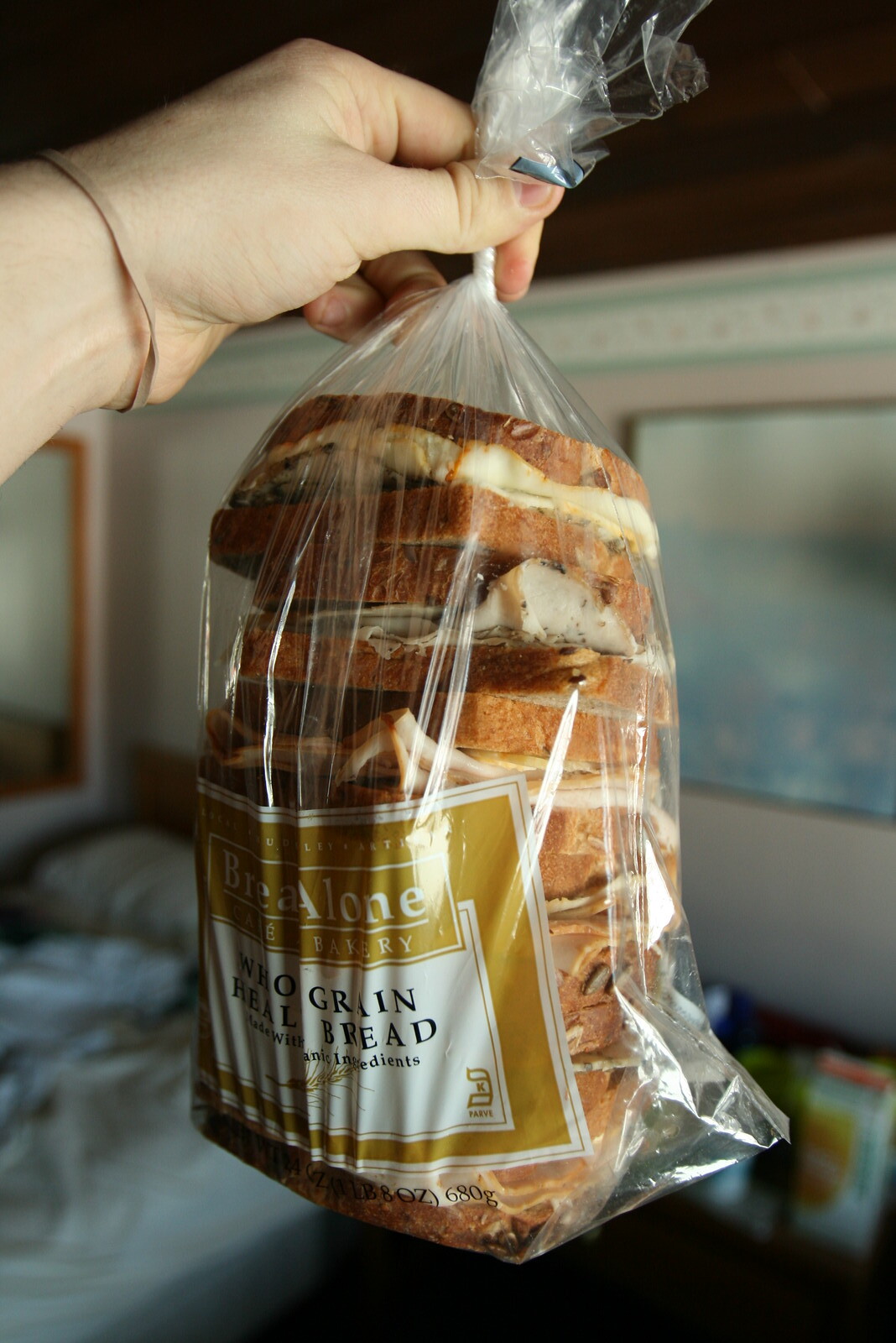In this image, taken indoors with a very blurred background, a person with a Caucasian hand is holding a plastic bag containing several sandwiches. The hand, which has a rubber band on the wrist, appears to pinch and twist the top of the bag to seal it shut. The bag is labeled with partially visible text, including words like "bakery," "whole grain," and "real bread," and weighs 680 grams. The gold label features white and black lettering. Inside the bag, multiple stacks of sandwiches are visible, primarily made of ham between slices of bread. In the out-of-focus background, a messy bed is noticeable on a pink wall, along with blurred images of water and mountains, a mirror, and some pantry goods on the floor.